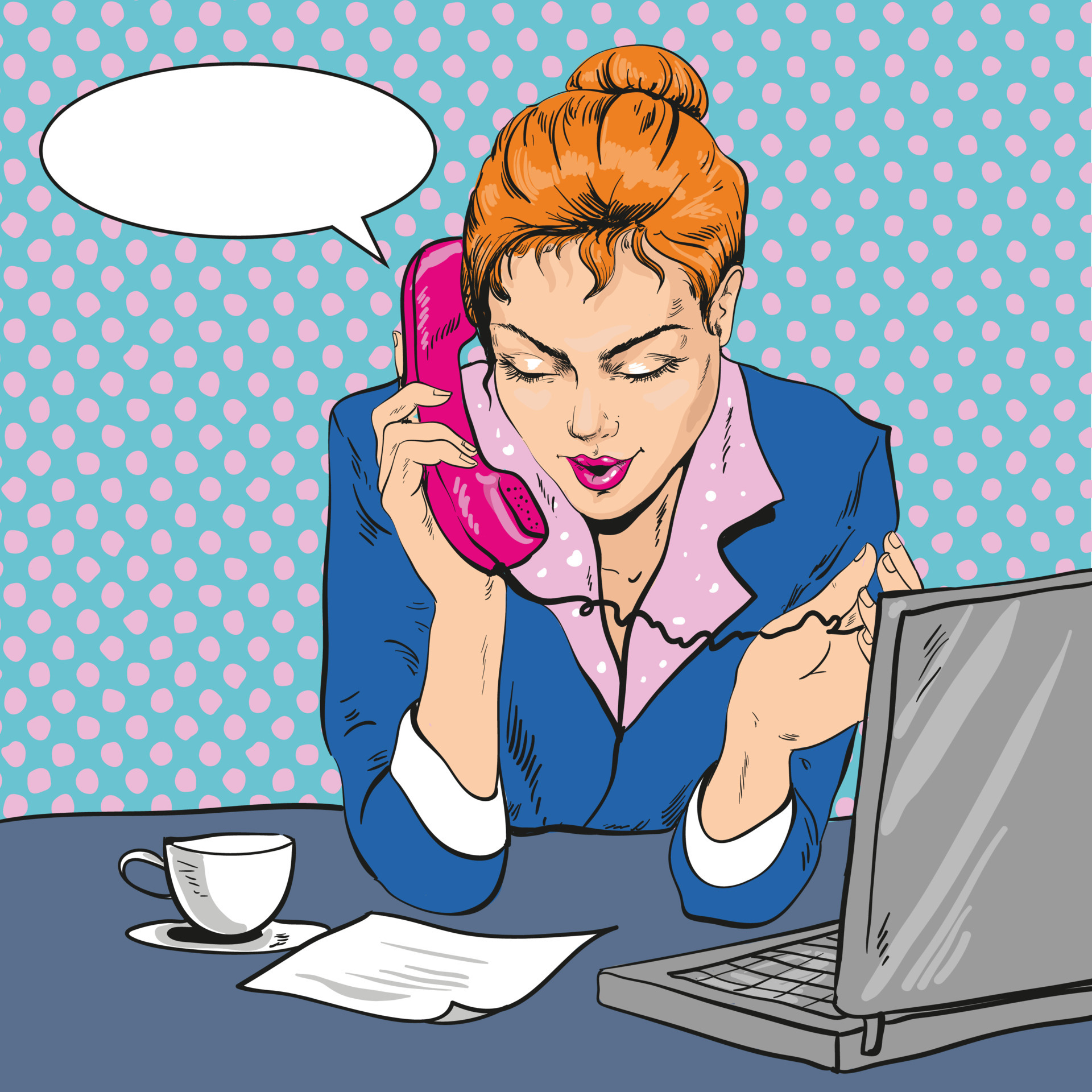The image is a retro-style digital art piece, likely resembling a comic book still. It features a woman with light beige skin and striking red hair piled in a bun, her head tilted down as she talks on a bright magenta, Barbie-pink phone with a black cord. Her lips share the same vibrant hue as the phone, enhancing her animated appearance. Dressed in a blue jacket over a pinkish shirt with a lavender-colored collar, she rests both elbows on a bluish-gray desk. On the desk, to her right, sits an open gray laptop, and to her left, a piece of white paper and a white coffee cup on a saucer. The backdrop is a playful baby blue with pink polka dots, giving the scene a whimsical touch. There's also a blank white speech bubble emerging from the left side of the image, adding to the comic strip vibe.